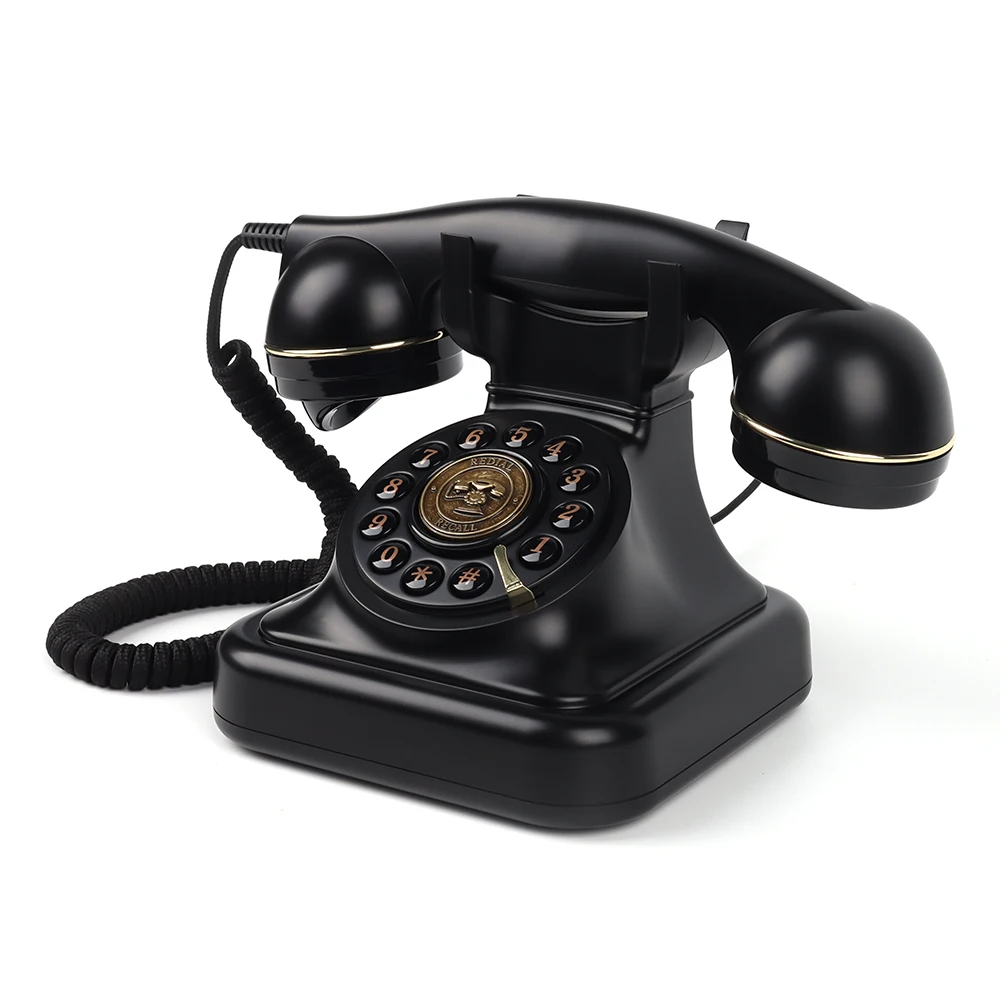This photograph showcases a black, retro-style rotary telephone set against a stark white background. Despite its vintage appearance, the phone exhibits a modern twist with push-in buttons replacing the traditional rotary dial. These glossy black buttons feature light brown numerals alongside an asterisk and a number symbol, nestled in the middle section of the phone. At the center of this dial area, a bronze-colored emblem displays an intricate, embroidered metal telephone icon, beneath which the words "We Dial" and "Recall" are inscribed. Crafted from plastic, the phone flaunts a sleek, modern aesthetic with a thicker, more contemporary-looking receiver. The coiled cord connects the receiver to the base, where it securely clicks into place without relying on the pressure-sensitive mechanism of original rotary phones. The overall design is completed with brushed nickel accents around the earpiece and mouthpiece, highlighting the handset's elegant, matte black finish.